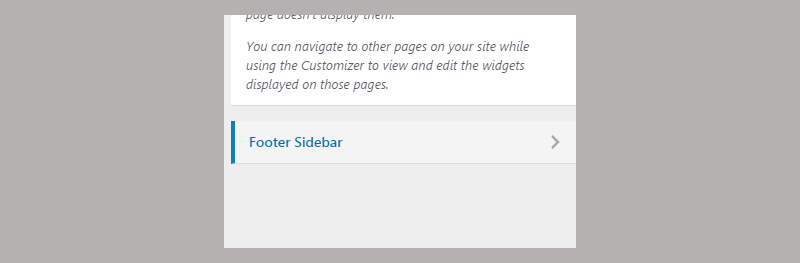The image is a cropped screenshot from a website or application, showcasing a very zoomed-in section. The entire shot is framed by a large gray border with the central content displayed on a gray background. The zoomed-in area is divided into two main sections: an upper white text box and a lower area with a gray background.

In the upper white text box, gray text reads: "You can navigate to other pages on our site while using the customizer to view and edit the widgets displayed on those pages." Below this text box, there is a slightly off-gray area featuring the phrase "footer sidebar" written in blue font. Adjacent to this phrase on the left is a small vertical blue line, suggesting a marker or separator. To the far right of this area, a gray arrow pointing to the right indicates an expandable or interactive element.

At the very top of the zoomed-in section, there is an additional line of text, but it has been cut off and is thus unreadable. The overall layout suggests it is a customizable interface within a web design or content management system.